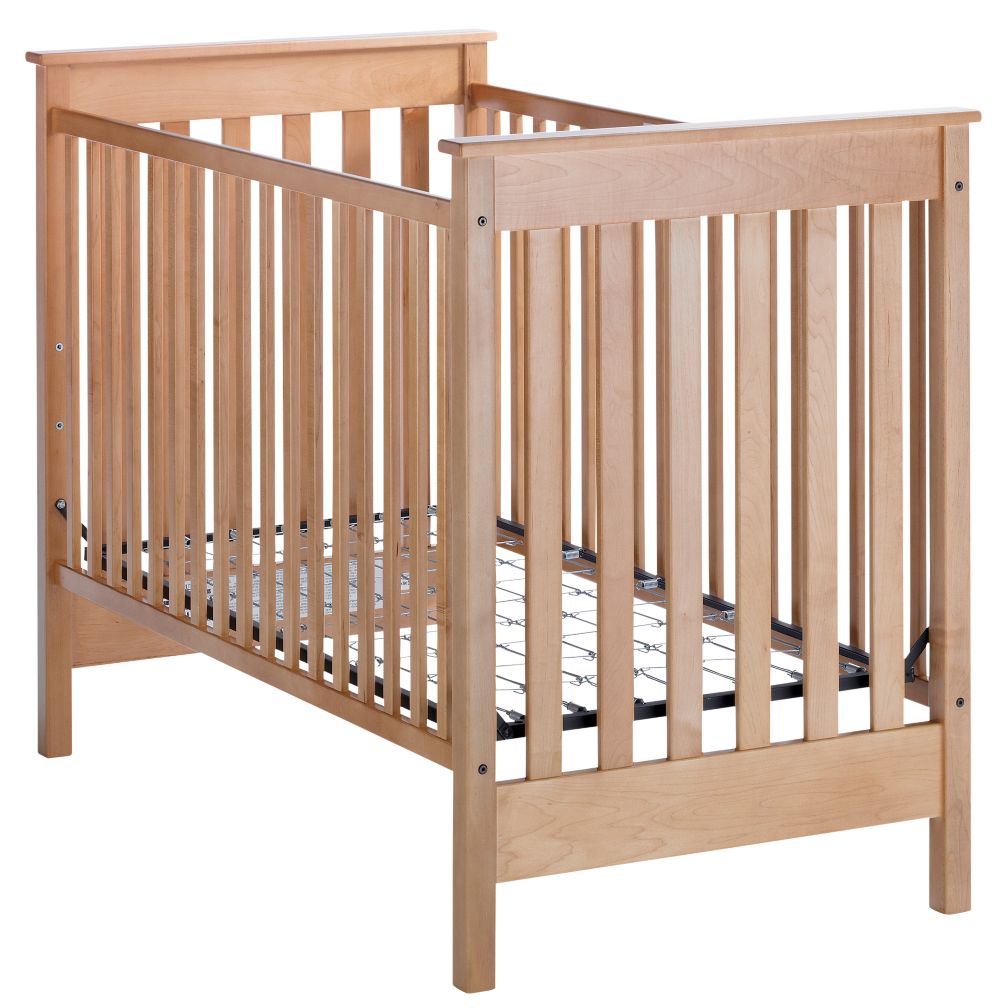This image showcases a light brown wooden crib, captured as a catalog product photo with a clean, edited background. The crib's design is minimalistic, featuring long strips of wooden slats arranged in a grid-like pattern. It stands on four legs, although only three are visible due to the isometric perspective. The structure is rectangular, and the headboard is positioned to the right while the sideboard extends to the left. Inside the crib, there is no mattress, but a black metal spring foundation, which has silver netting for mattress support, is visible. The crib is fully assembled and displays visible screws at the front and back.